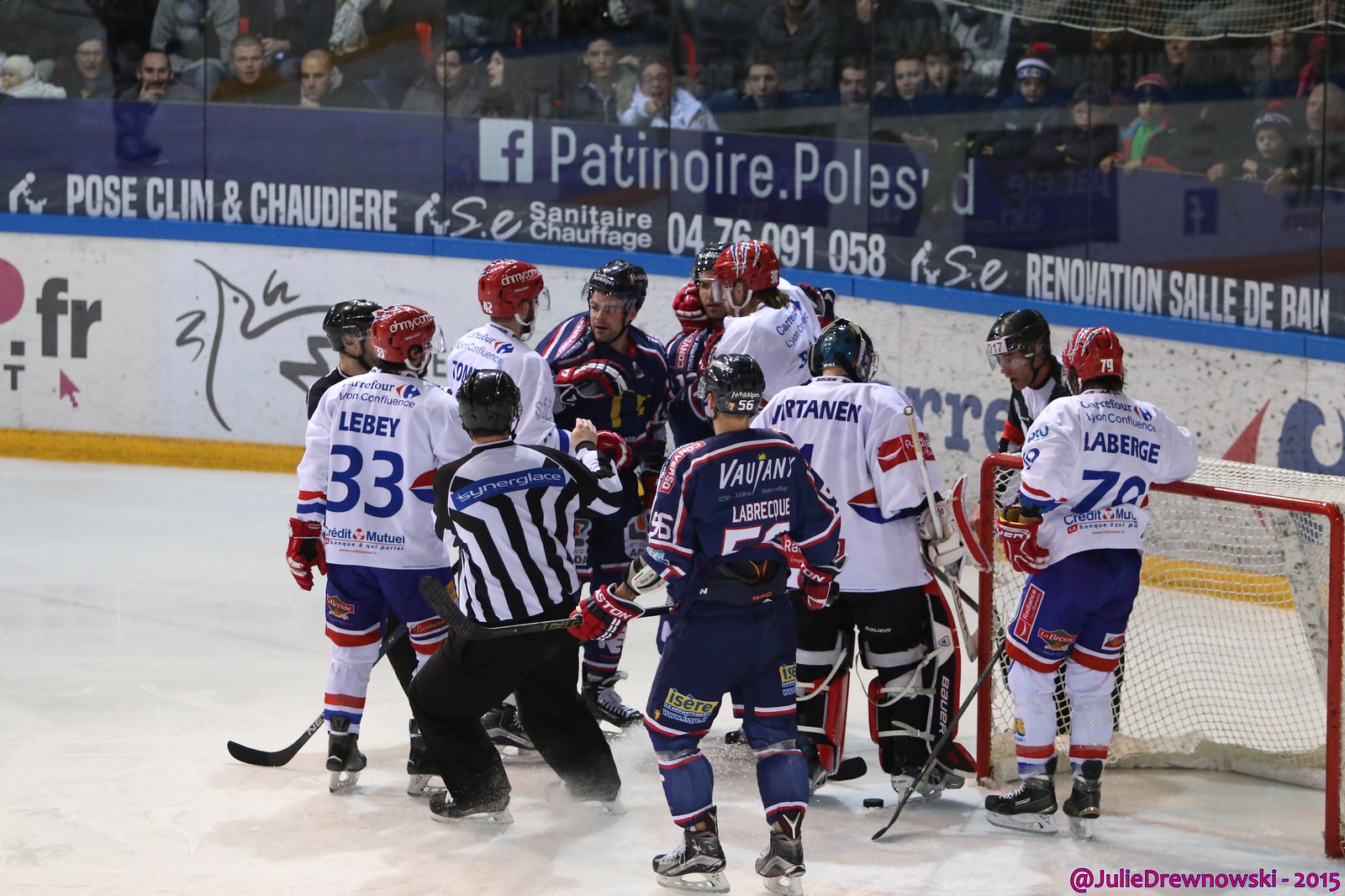This indoor color photograph captures an intense moment during an ice hockey game in a sports stadium. The scene is dominated by a group of players from two teams, one wearing blue jerseys and the other in white, who appear to be involved in a skirmish around a single spot on the ice, likely where the puck is located. A referee is present, attempting to mediate the situation. The background, separated from the action by a plexiglass barrier, is filled with numerous spectators, predominantly men, who are intently watching the game unfold. Various elements of the arena are visible, including the net, hockey sticks, and the rink itself, enclosed by glass. Advertisements in French, including one for Carrefour, and other French text like "Patinoire" and ".fr" suggest the game is taking place in France. Brightly colored details such as red, white, blue, black, green, orange, and a fuchsia hue add to the vibrancy of the scene. In the bottom right corner of the image, the photographer's credit "at Julie Drunowski 2015" is visible. This photograph perfectly encapsulates the dynamic and spirited atmosphere of an ice hockey match.